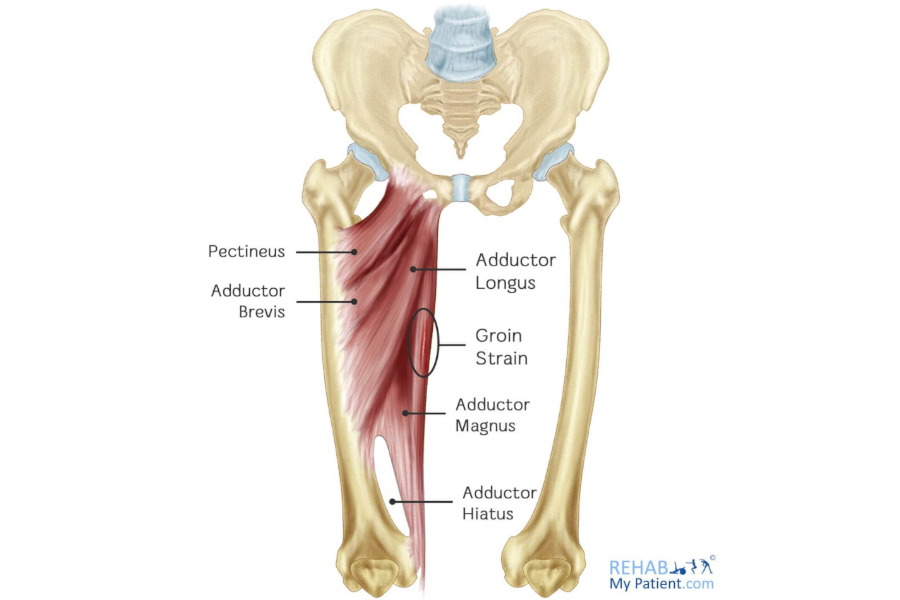This detailed medical diagram, sourced from rehabmypatient.com, illustrates the male hip and upper thigh from a coronal or forward-facing view. It prominently features both the skeletal structure and specific muscles relevant to groin strains, depicted in shades of pink and blue against a plain, background-free backdrop. Key anatomical labels include the pectineus, adductor brevis, adductor longus, adductor magnus, adductor hiatus, and a marked area indicating a groin strain circled in black. This educational illustration spans from the pelvis and hip bones down to the top of the knees, effectively highlighting the inner complexities and connections of these regions. The diagram is user-friendly for those undergoing rehabilitation, seeking to understand specific muscles affected by groin strains, and the source website is credited in blue text at the bottom right corner.